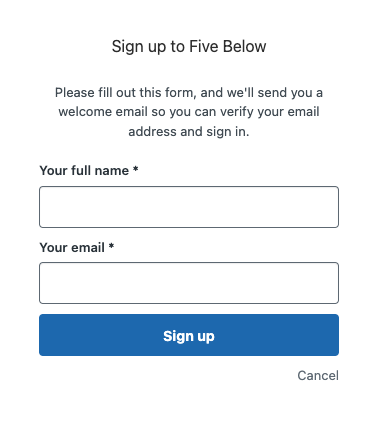A white background features a user registration form with various text elements and input fields. At the top, black text reads, "Sign up to find below. Please fill out this form, and we'll send you a welcome email so you can verify your email address and sign in."

Below this, a white rectangular input box labeled "Your full name" is present, where only the first letter of the first word is capitalized. Underneath this input box is another labeled "Your email," also in black text.

At the bottom of the form are two rectangular buttons: a blue one labeled "Sign up" with a capital 'S' and lowercase 'u,' and a white one labeled "Cancel" in the bottom right corner.

The entire form is set against a simplistic white backdrop, emphasizing the straightforward and minimalistic design intended for user ease.